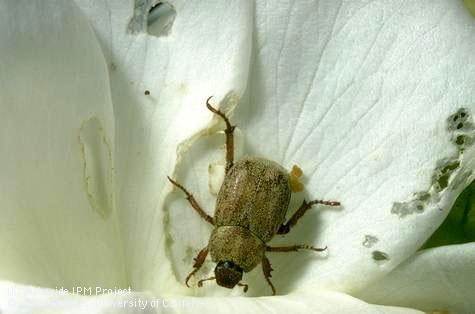The detailed, close-up image features a beetle on a white flower petal, showing intricate details of both the insect and the petal. The beetle has a tan and speckled brown body, with a round shape, and a tiny black head adorned with short antennae. Its six legs are clearly visible, with the back legs being the longest—one of which is extended backward. The insect appears to be situated towards the bottom middle of the image, facing downward. Surrounding it, the flower appears diseased, with noticeable holes and a large chunk missing, bordered by green and brown discoloration. Three overlapping petals form the background, and there is some barely discernible white text along the left side, containing words like "project", "IPM," and "university." Despite some confusion in initial observations about the background being a napkin or paper towel, it is discernible that the beetle is on a flower petal. The meticulous close-up captures the damaged petal in striking detail, contributing to an overall sense of decay or disease affecting the flower.